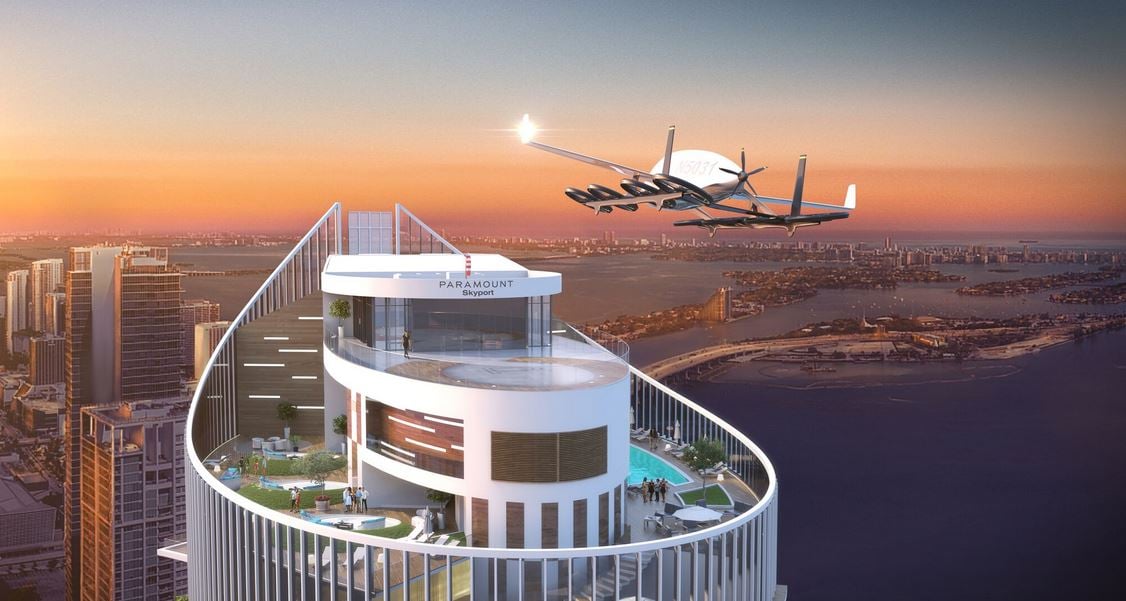The image is a computer-generated, wide, horizontal rectangular drawing depicting a futuristic cityscape, reminiscent of Miami, set against a breathtaking sunrise or sunset sky filled with hues of pink, orange, and blue. The centerpiece of the image is an ultra-modern high-rise with the topmost area emblazoned with the word "Paramount Skyport." This building features a teardrop-shaped structure composed of white metal rods forming vertical, oval patterns that peak towards the back. 

At the top of the building, multiple levels are visible, including a lower level adorned with swimming pools, green grassy areas, and trees, providing spaces for people to gather and relax. Above this, a circular helipad is prominently displayed, prepared for aerial arrivals. A futuristic aircraft, a hybrid between a helicopter and a jet with eight wheels, white blades, and wings, is approaching for landing. 

In the background, numerous additional skyscrapers rise from islands connected by bridges, surrounded by expansive bodies of water, suggesting a coastal or beachside setting akin to a tourist hub like Florida. The glass railings around the building's perimeter add to the sleek and advanced aesthetic of the entire scene.